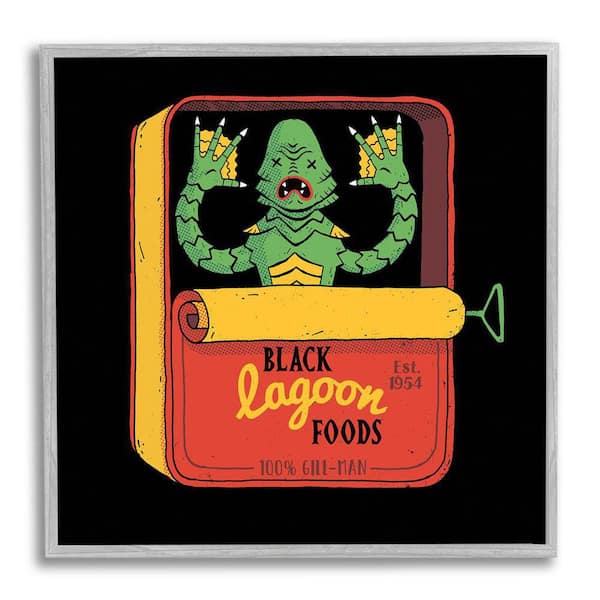The image is a detailed, framed art print set against a white background with a shadow cast to the bottom left. The frame is made of light grey wood. The artwork itself features a vivid green cartoon creature from the Black Lagoon with webbed fingers, yellow-tipped features, red lips, and X's for eyes. This creature is positioned in a half-open, old-fashioned metal tin or sardine can, colored in striking yellow and red. The can is partially unrolled with the help of a green key and has a label that reads "Black Lagoon Foods, EST 1954, 100% Gilman." The black background of the art print creates a dramatic contrast, making the central character and vibrant colors stand out, giving the whole piece an eye-catching appearance suitable for home decor or as a collectible art print.